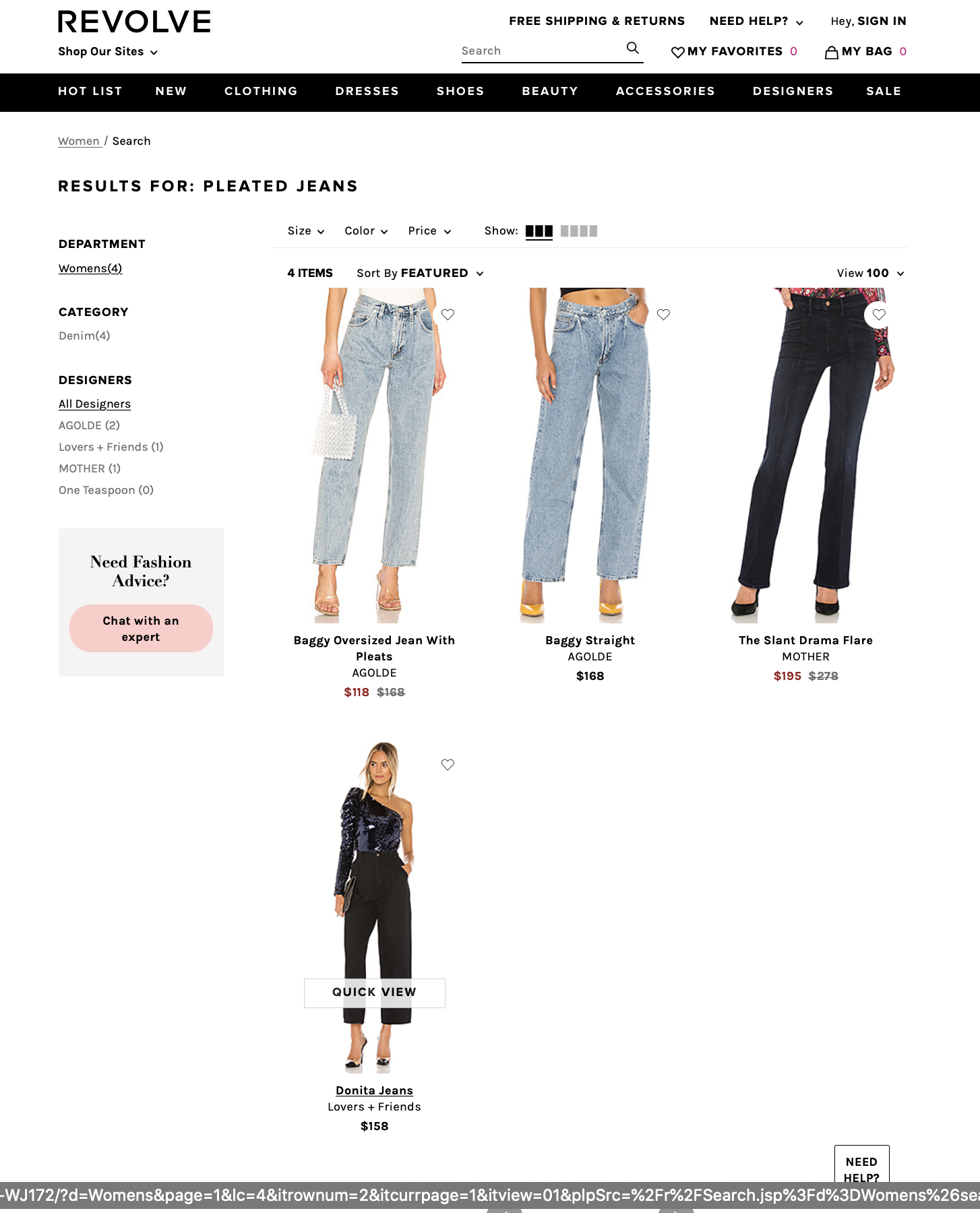Screenshot of the Revolve shopping website for women's clothing with a white background. 

In the upper right corner, features include "Free Shipping and Returns," a drop-down "Need Help?" menu, and a "Sign In" prompt.

The website's name, Revolve, prominently appears in large black font in the upper left corner. Below this is a drop-down menu labeled "Shop Our Site," a search field marked by a black line with a "Search" prompt in black font above it, and a black magnifying glass icon. Adjacent to the search field is a heart icon labeled "My Favorites (0)" and a bag icon labeled "My Bag (0)."

A horizontal black bar with white text provides navigation options: "Hot List," "New," "Clothing," "Dresses," "Shoes," "Beauty," "Accessories," "Designer," and "Sale." Below this bar, in gray font, it reads "Women / Search."

The search results section begins with the heading "Results for: Pleated Jeans," displaying four image results of jeans. The first selection is a pair of "Baggy Oversized Jeans with Pleats" priced at $118, featuring a stonewashed finish.